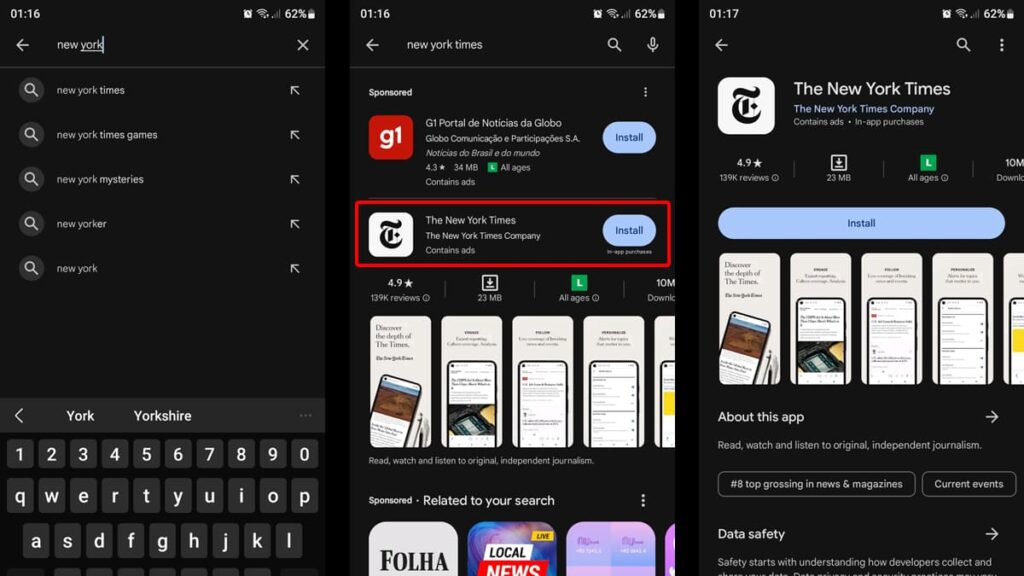The image depicts a side-by-side comparison of three web pages displayed horizontally. 

The first webpage, positioned on the far left, simulates the search interface on a mobile device. In the top left corner, there's a timestamp showing "01:16." The top right corner includes an alarm clock icon, Wi-Fi symbols indicating connection strength, a battery percentage display at "62%," and a padlock icon. Just below these elements, a left-pointing arrow in light gray is present, alongside a search bar with the text "New York," where the word "York" is underlined by a thin horizontal gray line. The search bar itself contains a horizontally displayed typing line. On the far right of the search bar, there's a light gray "X" for clearing the input. 

Below the search bar, a list of search suggestions is shown, each prefixed by a circular icon with a light gray magnifying glass. The suggestions include, from top to bottom: "New York Times," "New York Times Games," "New York Mysteries," "New Yorker," and "New York." Each suggestion is followed on the right side by a light gray arrow pointing to the upper left, signifying a subsequential link. At the bottom of this webpage, there's a horizontal gray bar that reads "York" and "Yorkshire," accompanied by an arrow pointing to the left and an alphanumeric keyboard.

The second webpage, in the middle panel, showcases a list of web pages. The highlighted item here is the "New York Times" installation of a web application, placed below the "Globo News Portal" application ("G1 portal de notícias de Da Globo").

The third webpage, positioned on the far right, is the installation page for the "New York Times" application. This page exhibits example panels demonstrating what the app's interface looks like. Beneath these panels is a prominent, long, light blue, pill-shaped button labeled "Install."